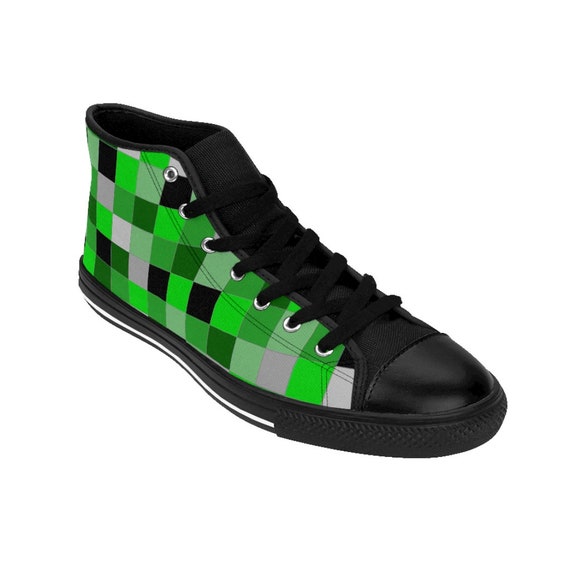This image features a computer-generated clip art of a high-top sneaker against a white background. The sneaker has a distinctive and colorful design, with a body covered in a checkered pattern of light green, dark green, black, and occasional white squares. The sneaker has a shiny black tip that rounds off at the front, transitioning into a black canvas or similar material for the upper part. The shoe is equipped with black laces threaded through seven eyelets. The black sole is bordered by a white line that follows a slightly wavy band around the edge. 

The image contains no text, focusing solely on the detailed and vibrant depiction of the sneaker.